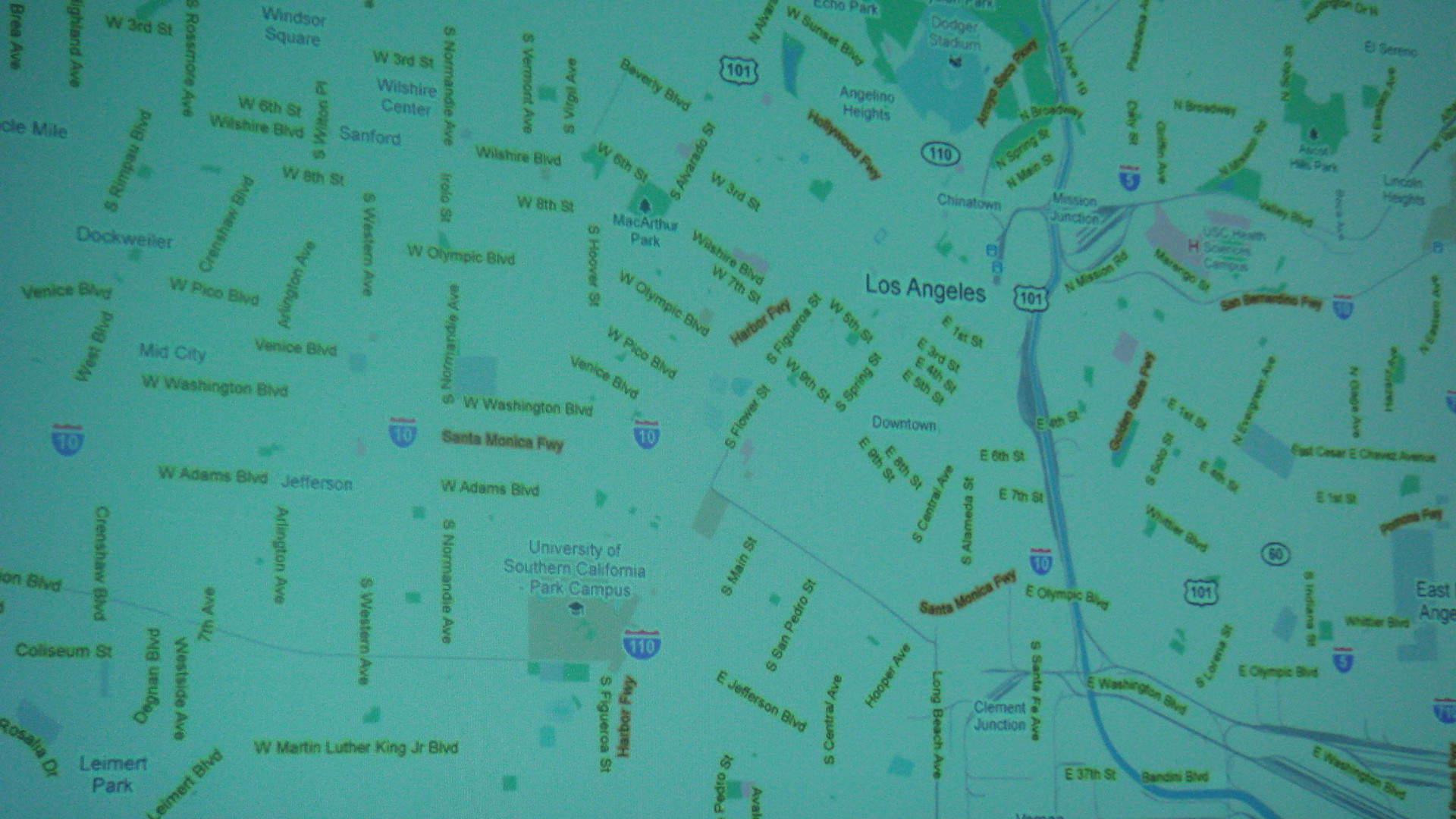A small turquoise blue square fragment of an indistinguishable map. The diminutive scale renders most text illegible. A darker blue waterway is discernible on the right side, stretching diagonally from the bottom right to the top right corner. The remaining visible elements consist of faint, mostly unreadable labels set against a light greenish background, suggestive of various streets, roadways, and other geographic features. Certain text elements appear slightly bolder, possibly indicating larger towns. The image resembles a map viewed from a significant height, presenting an array of angled, horizontal, diagonal, and vertical lines representative of labeled paths. Scattered across the map are heart-shaped blue, white, and red U.S. interstate signs, but their numbers are unreadable. No distinct markers indicate the geographic area depicted, with the absence of identifiable city names or specific region labels.